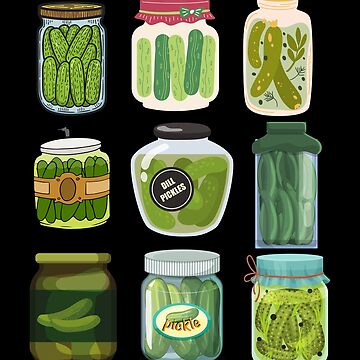This is a detailed graphic art piece showcasing nine hand-drawn pickle jars, arranged in a 3x3 grid against a pitch-black background. Each jar features distinct characteristics and artistic styles, emphasizing the diversity of pickle presentation. The top row includes a mason jar with a cork lid and green pickles, a wider mason jar with a red top, and a beige mason jar with a small lid. The middle row starts with a wider jar with a white cap and a brown label, followed by a large jar with a black top labeled "dill pickles," and a tall jar with a green cap. The bottom row consists of a store-bought-looking jar with a yellow lid and a pickle label, a jar with a white lid labeled "pickle" on a sticker, and a homemade-looking jar with a blue wrapper and a red ribbon tied around it. The jars vary not only in form and lid styles but also in the detailing of their contents, from fully packed to sparsely filled, indicating a collaboration of different artistic hands.